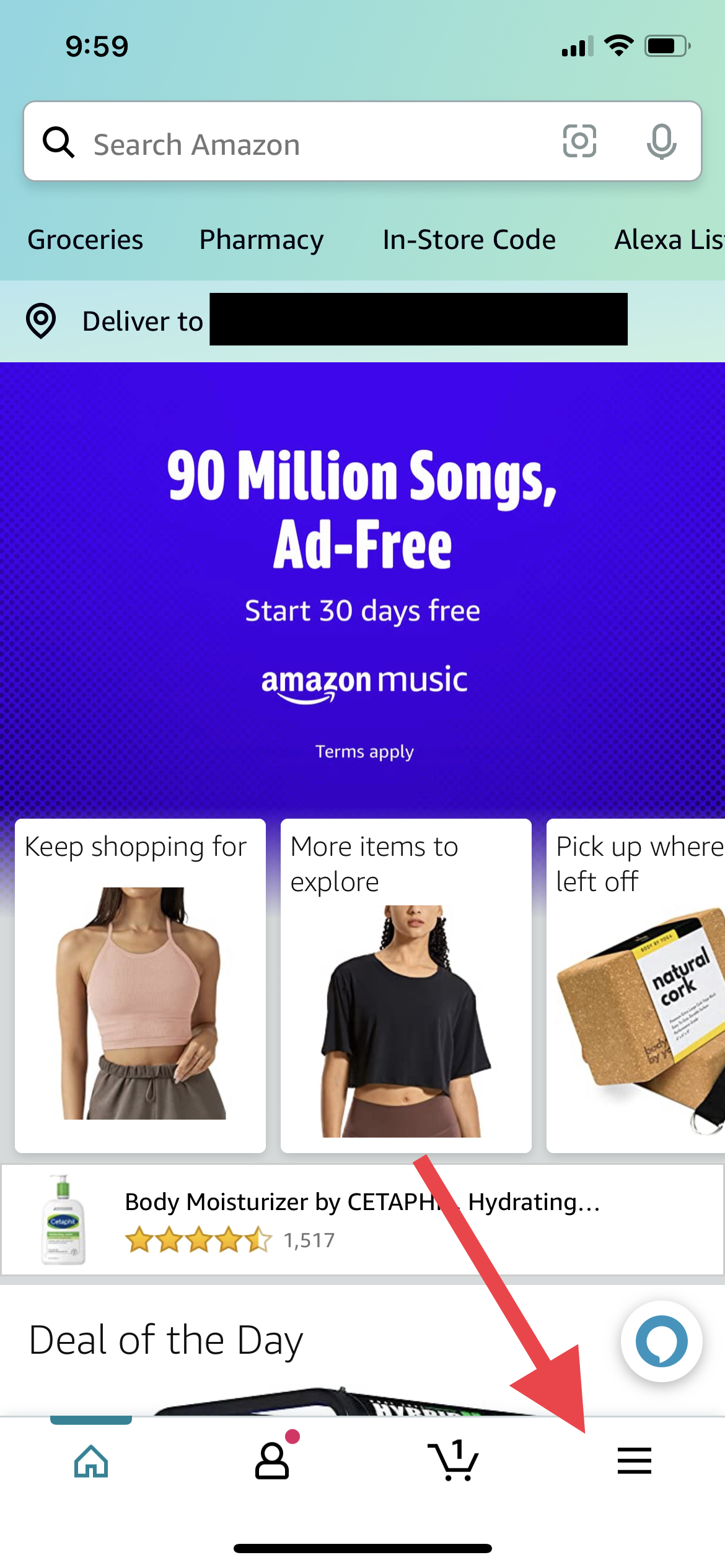This is a screenshot of the Amazon homepage taken from someone's phone. 

At the bottom of the screen, there are four navigation options: Home, Account, Cart, and More. The Home icon is highlighted in a blue-teal color, indicating it is currently selected, while the others are displayed in black. A notification badge, represented by a small red circle, is visible above the Account icon. A red diagonal arrow points toward the "More" categories option, accompanied by a speech bubble marking the way to connect with customer service.

The "Deal of the Day" section is partially visible but cut off, making it unclear what the specific deal is. To the left of this section is a suggested product - Cetaphil Hydrating Body Moisturizer. The product has a rating of 4.5 stars based on 1,517 reviews, with an image of the moisturizer displayed to the left of the rating.

Above these suggestions are three boxed options: "Keep shopping for," "More items to explore," and "Pick up where you left off," each with corresponding pictures of items the user might be interested in or has previously viewed.

Further up, a blue banner advertises "90 million songs ad-free" with Amazon Music. Below this message, there is a prompt to "Start 30 days free," followed by the Amazon Music logo and a small-font note stating "terms apply."

At the very top of the screenshot, the phone's status bar shows the time, cellular reception, Wi-Fi status, and battery life, all set against a bluish background. Below this, a white search bar labeled "Search Amazon" allows the user to either type, speak, or take a picture for their search query. Underneath, a blue background features quick-access options for Grocery, Pharmacy, Store Code, and Alexa. An option starting with "LIS" is partially visible and likely cut off.

Finally, the location symbol indicates "Deliver to," but the specific address information is redacted, presumably for privacy reasons.